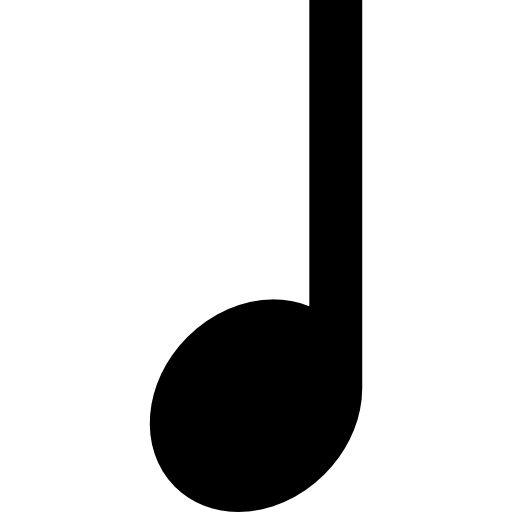This image is a detailed, large, black musical note positioned against a stark white background. The note resembles a lowercase "D" with its bottom part being a solid black, rounded shape, and the upper part extending into a long, thick rectangle that tilts slightly to the right, likened to the end of a golf club or a stick. The simple, clean composition emphasizes the high contrast between the black note and the white backdrop, allowing the viewer to focus solely on the note. The image has no edges visible and is likely a clipart due to the lack of additional elements or colors, giving a clear, isolated representation of the musical note in a black-and-white, illustrative format.